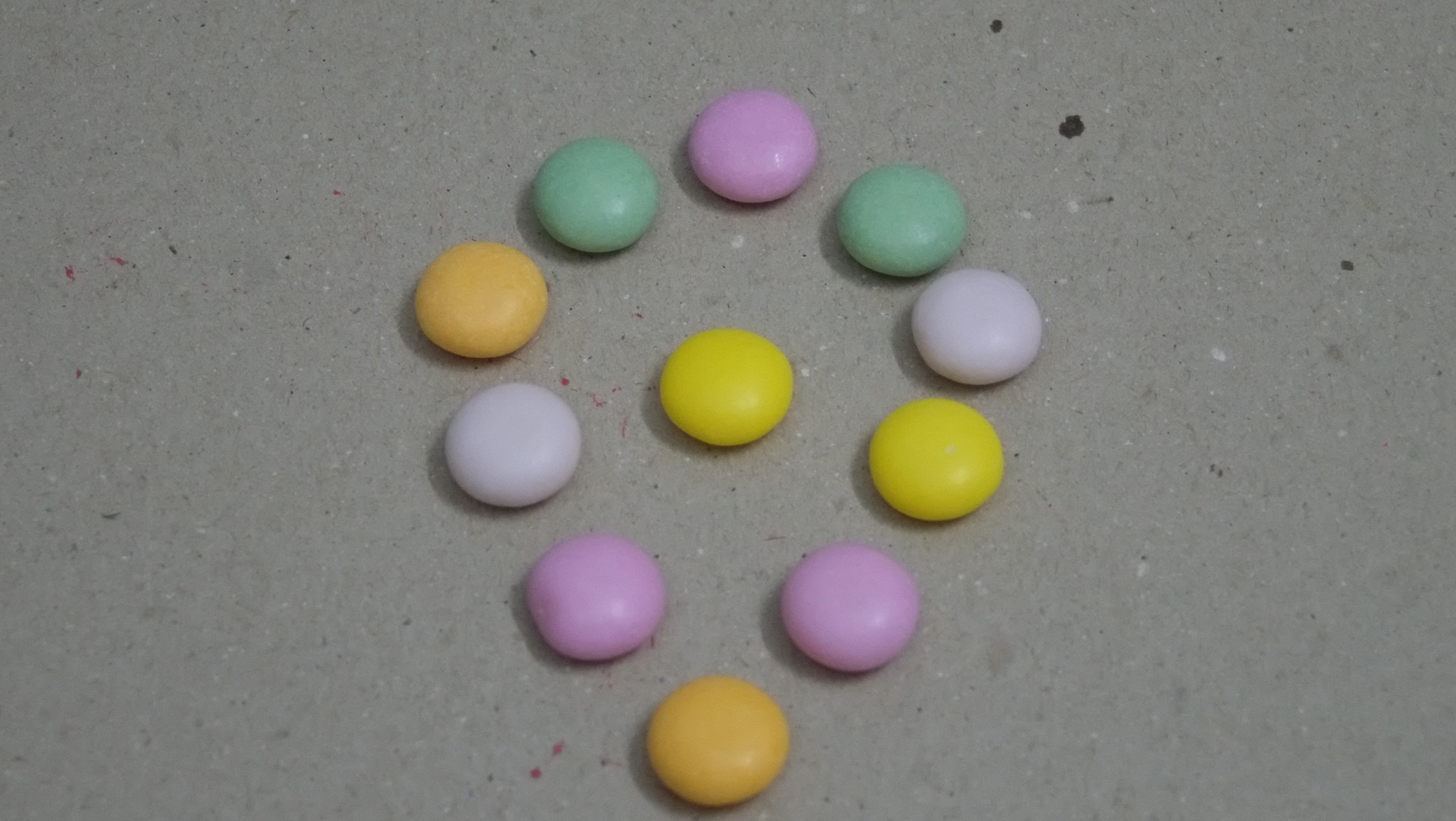The photograph features 11 pastel-colored coated mints closely resembling M&Ms or Smarties, arranged in an inverted teardrop shape with the rounded part at the top and the point at the bottom. The colors of these mints include pale green, pink, light orange, light purple, lavender gray, and yellow, with a yellow mint positioned centrally within the teardrop shape. These small, round candies are placed on a grayish background, likely resembling construction paper or cardboard, accented with darker gray, red, and black dots scattered throughout. No text or additional context is provided in the image to convey further information.